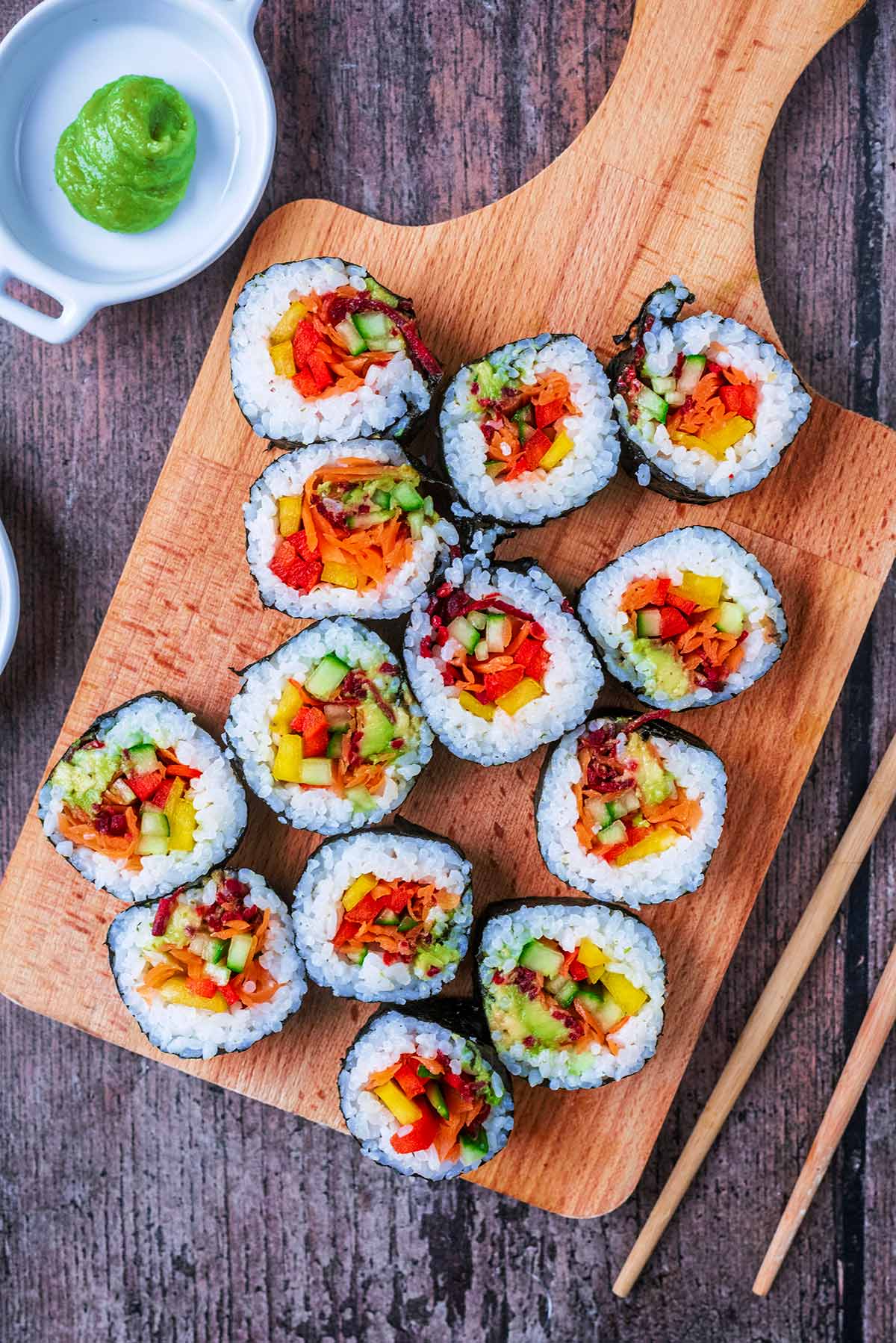This detailed portrait-oriented photograph showcases a wooden background with lateral striations in a reddish-brown hue, resembling a sun-bleached wooden surface. Centered in the image is a light tan rectangular cutting board with a handle pointing to the upper right. Positioned on the cutting board are 13 neatly arranged pieces of sushi, each wrapped in seaweed with a rice outer layer. The colorful interiors are visible, featuring a variety of vegetables that include shades of yellow, green, red, and orange, possibly carrots, squash, and tomatoes. To the right of the cutting board, a pair of chopsticks rests on the wood surface. In the upper left-hand corner, there is a white circular bowl containing green wasabi, and nearby, only the rim of another white bowl is visible.